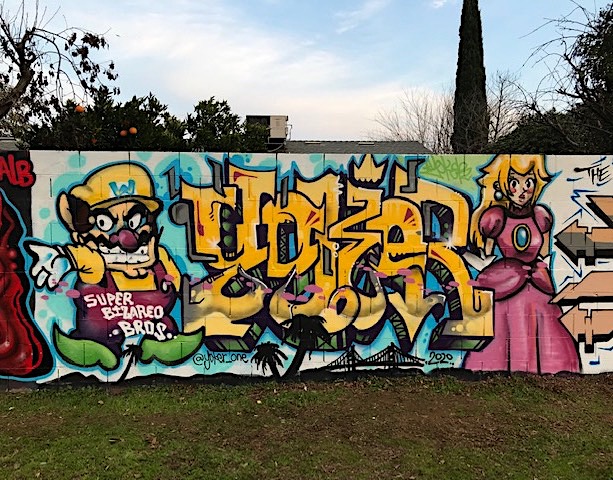The image depicts a colorful and detailed graffiti mural on a cinder block wall, illuminated by daylight. On the far left, there is a distorted version of Mario from Super Mario Bros., characterized by a yellow cap with a blue 'W', a large red nose, a gloved white hand, a yellow shirt with red overalls, and green shoes. The overalls sport the phrase "Super Bizarre Bros." in white. In the center of the mural are stylized, three-dimensional letters in yellow, which appear to spell "U.D.B.Z.E.R." To the right is a reimagined version of Princess Peach, donning a red gown decorated with a blue jewel and her signature blonde hair. Several brown arrows point towards her, and the numbers "2020" are inscribed to the bottom left of her figure. Additionally, there is a simple black drawing of a bridge to the left of the princess, flanked by two black palm trees and an indecipherable signature. The wall is surrounded by grassy terrain, with some patches appearing worn. In the background, there is a house partially obscured by foliage, including an orange tree and treetops. The scene is set against a backdrop of a minimal sky with some cloud cover.